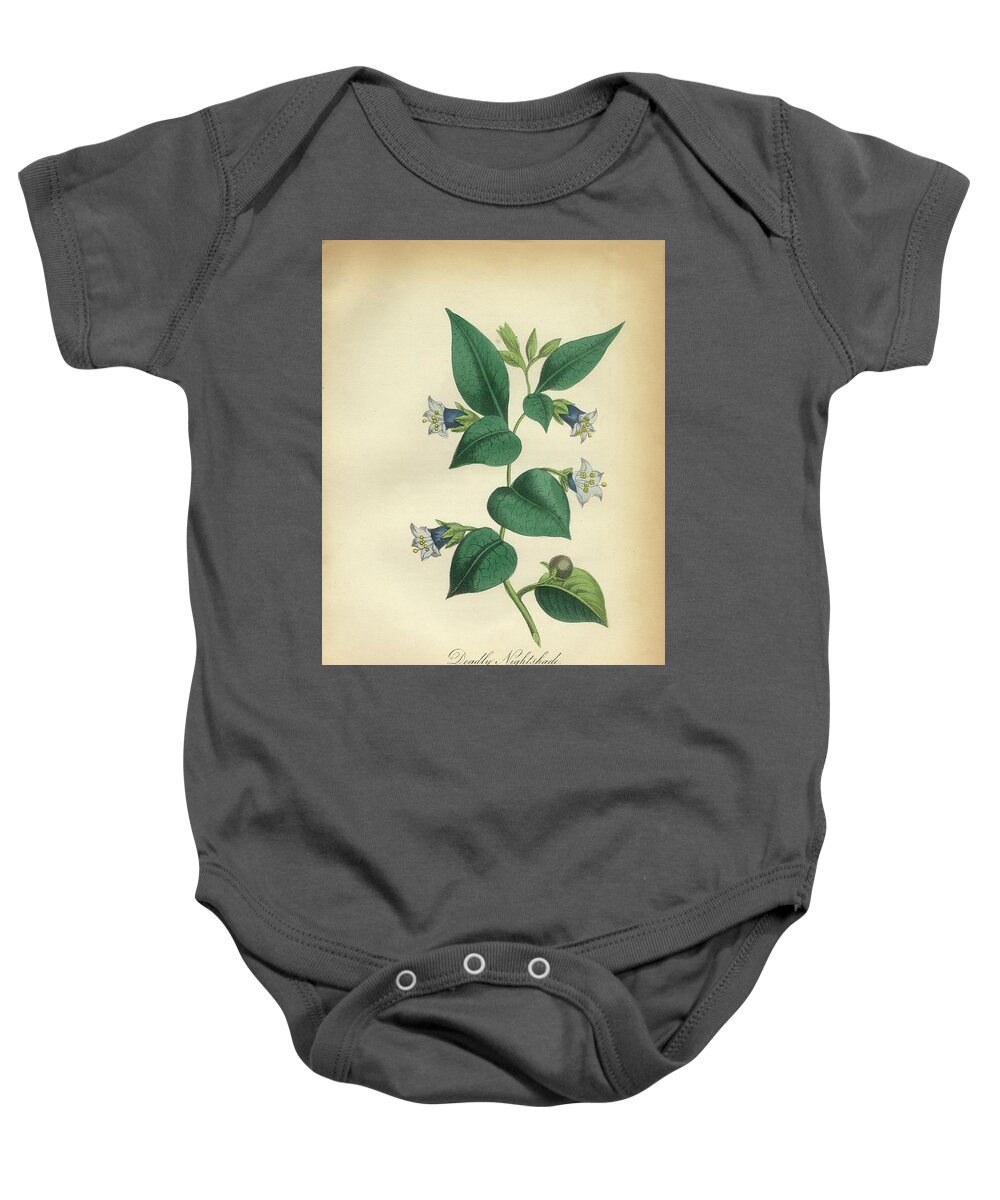This image showcases a dark charcoal gray, short-sleeved baby onesie, designed without legs, and featuring three silver snap buttons at the crotch area. Displayed against a white background, the onesie prominently features a vertical rectangular image on its chest. The artwork has a background that is gold or beige, presenting a vintage painting of a plant with various shades of green, heart-shaped leaves. Among the foliage, there are small clusters of bell-shaped white and blue flowers, complete with yellow stamens. A closer inspection reveals a small brown and green snail nestled on the bottom-most leaf.